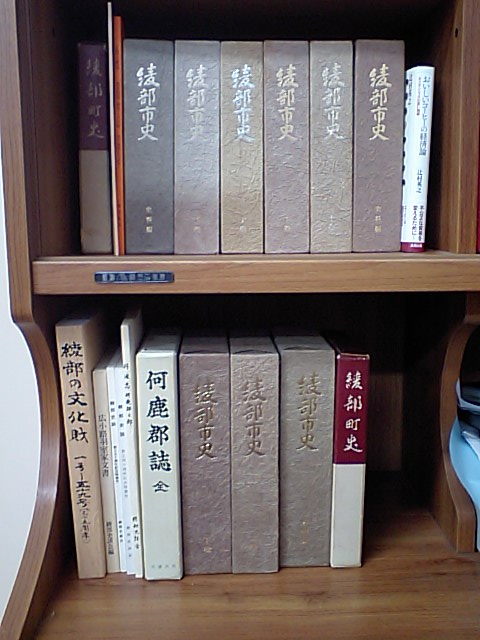A vertical rectangular photograph showcases a brown wooden bookshelf with distinct wood graining, featuring two shelves filled with an array of books. On the top shelf, six uniform books, aged and shaded from black to brown with silver Japanese or Chinese writing on their spines, dominate. To the left of these, there's a book with a purple top half and a tan bottom half. Next to it is a white and orange pamphlet-style book. On the right, there's a distinctive white book with a red bottom section. Below these, a black tag with silver writing is visible. The second shelf displays a similar pattern with several more books. Three of these books match the grayish, silver-tone ones from the top shelf, continuing their series. Additionally, there are books with white and black writing and tan covers. At the far end of this shelf is a two-tone burgundy and white book. A blue object is visible just past these books, adding a pop of color to the otherwise neutral palette.